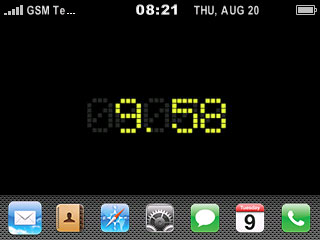The image depicts a smartphone screen with several visual elements. The upper portion of the screen is predominantly black, displaying essential status bar icons in white: full signal coverage, indicated by bars next to "GSM," the current time "08:21," the date "Thursday, August 20th," and a fully charged battery icon. Below this, prominently centered against the black background in gold numerals, the time "09:58" is shown, with the gray outlines of the zeros faintly visible.

At the bottom section of the screen, various app icons are arranged. These include a blue icon featuring a white envelope, commonly representing an email app, and an orange icon with a small brown figure, possibly a social media or messaging app. There is also an app for navigation, signified by a directional icon, and a calendar app distinguished by its red top and the number "9" within. A phone app with a green background displays a white handset icon. Additional apps are present but not individually described. The overall layout and icons suggest a standard home screen of a smartphone, organized for easy access to frequently used applications.